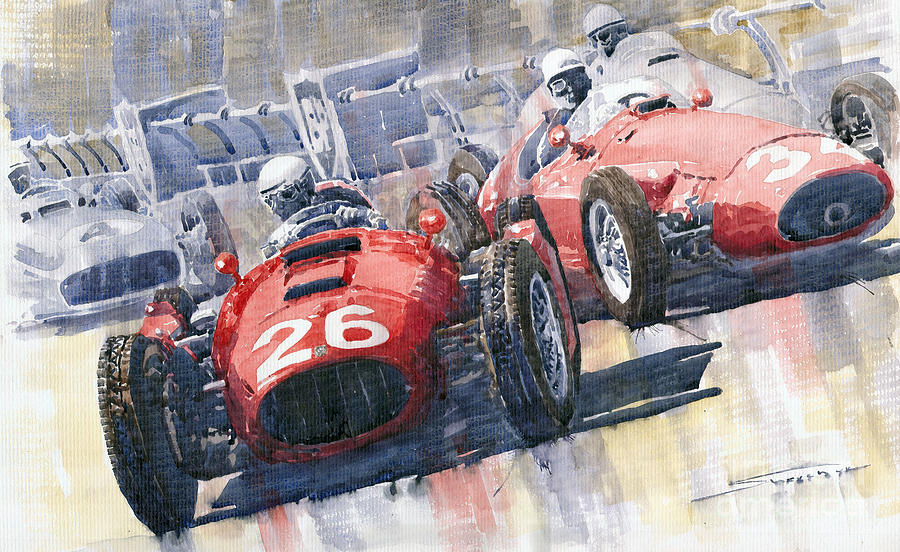The artwork captures the essence of a nostalgic 1950s Formula One race with a vivid, abstract interpretation. Dominating the scene are two prominent red race cars; the front-most car proudly displays the number 26, while the one to its right bears the number 34. The drivers are prominently visible, sporting white helmets with black goggles, characteristic of the era. 

Behind them, several gray race cars, less detailed and more abstract, fade into the background, creating a sense of depth and a contrast between the focal point and the subdued backdrop. Among these, a car numbered 4 can be discerned towards the top left corner. 

The painting's background is a swirling mix of vibrant reds, yellows, and whites, enhancing the overall dynamic and somewhat surreal quality of the scene. The textured ground similarly features an intertwining blend of blues and reds. Despite the cars appearing poised for motion, the artistic style renders them mysteriously stationary. 

In the bottom right corner, a signature is present but indecipherable, adding to the enigmatic charm of the piece. This horizontal artwork thus beautifully melds the thrill of vintage racing with abstract expressionism.